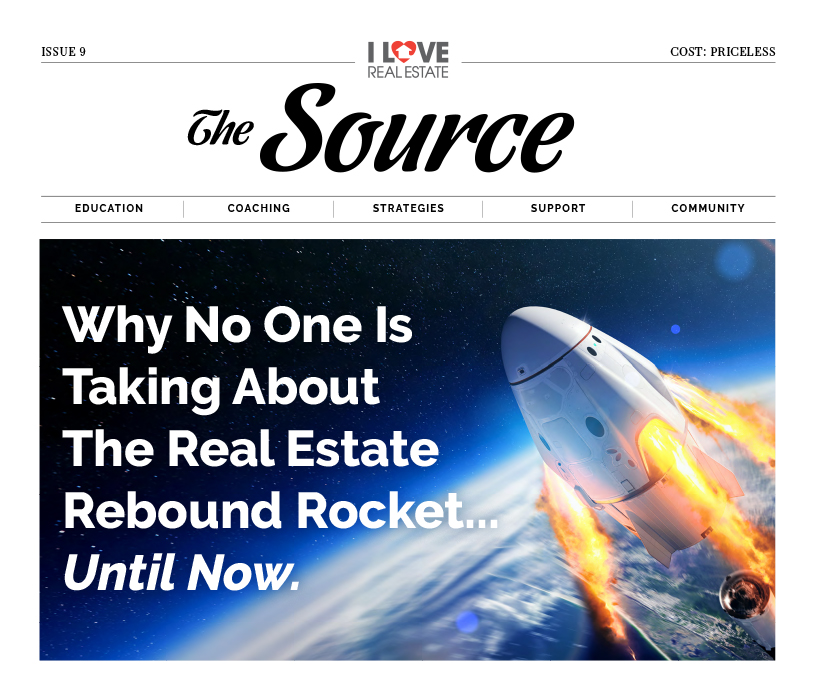In the image, we are presented with a visually engaging screenshot set against a solid white background. In the upper left corner, black text prominently displays "Issue Nine." Dominating the center of the image, the phrase "I Love Real Estate" is boldly written, with a heart adorned with an arrow substituting the "O" in "Love." Positioned in the upper right corner, the word "Priceless" indicates the cost.

Directly below this main header, a bold text segment introduces the source categories, reading from left to right: "Education, Coaching, Strategies, Support, Community." Beneath these words lies a striking, digitally rendered rectangular image of a spaceship. This spaceship, depicted in silver with dynamic flames trailing from its back, seems to be launching from the lower right corner. The lower portion of the image features the curved expanse of Earth, showcasing whites and blues with visible cloud formations encircling the planet. In the lower right, a blue area prominently displays the text: "Why No One is Talking About the Real Estate Rebound Rocket Until Now" in bold, white font.